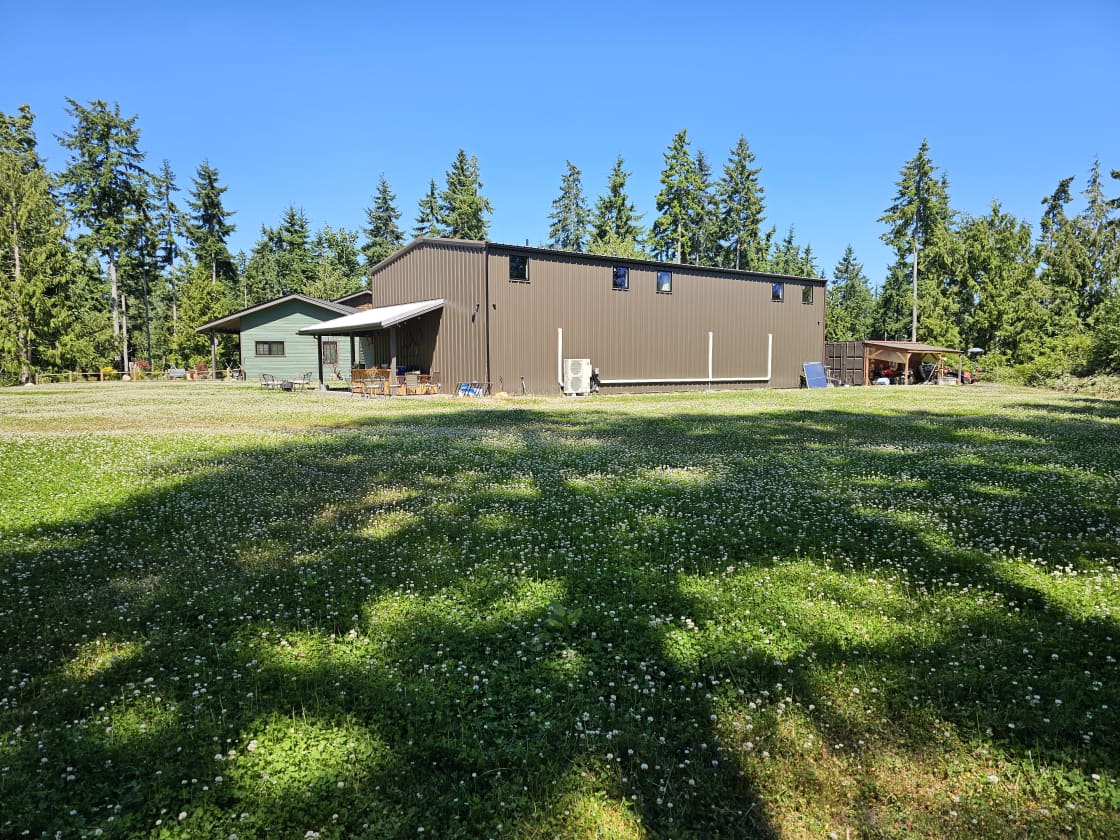The image depicts a serene scene of a vast green field, dotted with tiny white flowers, under a brilliant, cloudless blue sky. The field, bathed in sunlight, is marked by the dappled shadows of trees, indicating their presence behind the viewer. This sunlit pasture stretches towards the back, where a row of tall, verdant evergreen trees forms a natural boundary. Nestled among these trees, slightly in the distance, is a cluster of buildings. Dominating the scene is a brown, warehouse-like structure with small, high-set windows along its length and a front porch accented by an awning and bricks. Adjacent to this, on the left, stands a modest seafoam-green, one-story house, its charm enhanced by curtained windows. To the right behind the warehouse, a lean-to storage shed peeks out, completing the rustic tableau. This idyllic landscape captures the essence of a bright, tranquil day in the countryside.